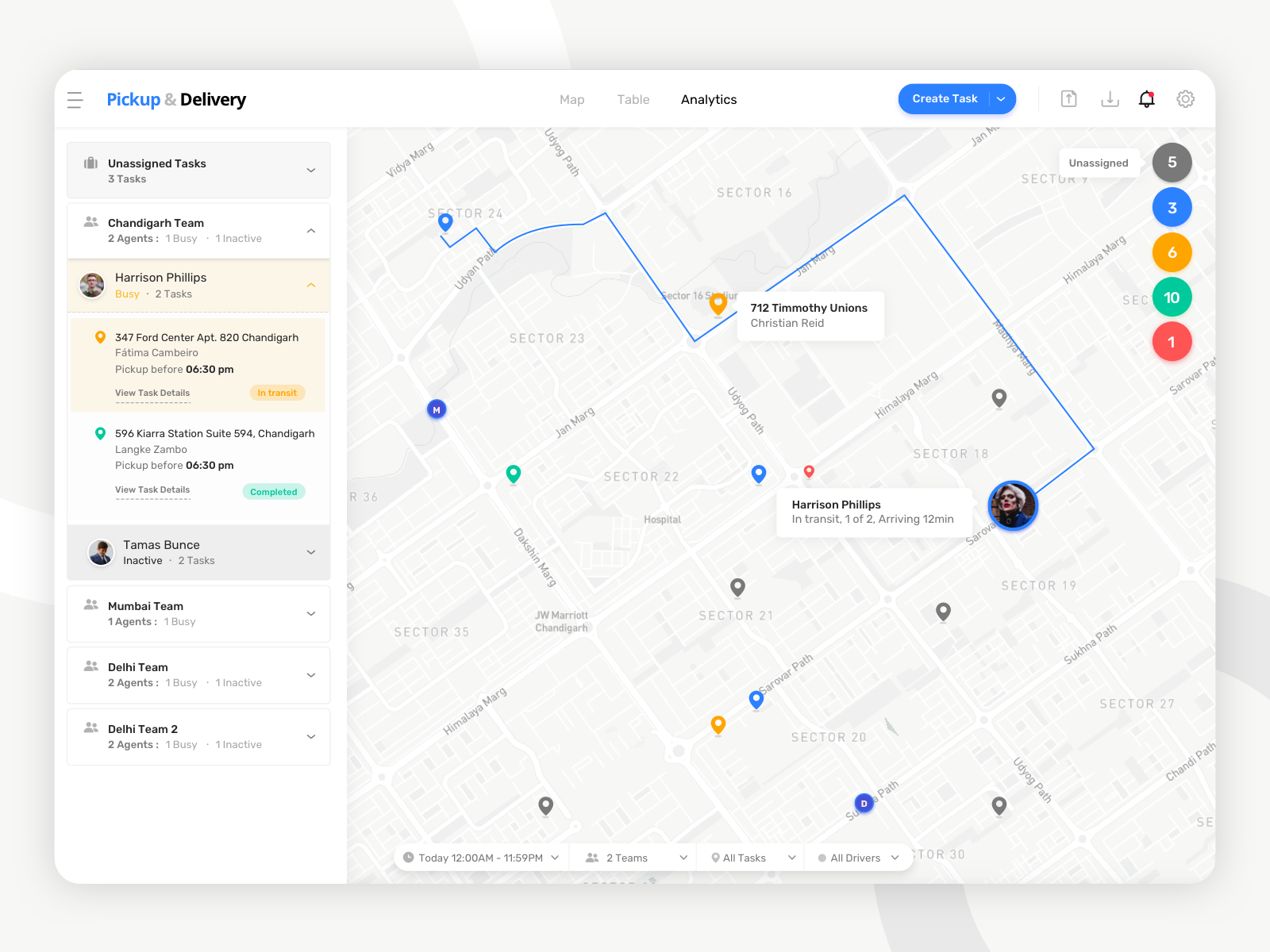In this screenshot set against a light gray background, we see a white interface screen prominently displayed. 

- **Upper Left Corner**:
  - In blue text, it reads "Pickup," followed by bold black text that says "Delivery."
  
- **Upper Section**:
  - To the right, there is a horizontal menu bar with items labeled: "Menu," "Map," "Table," and "Analytics" in black text.
  - On the far right, there is a button labeled "Create Task" in white text, and next to it, a blue button with a pull-down arrow.
  
- **Main Section**:
  - The main display features a map that is primarily light gray with white roads. Highlighted on the map is a blue line outlining a specific route.
  - In the upper left section of the map, there is a blue pin marking a location within areas referred to as Sector 23 and Sector 16.
  - Additionally, there is a red pin indicating "Harrison Phillips in transit," with a status note saying "one of two arriving in 12 minutes."
  
- **Upper Left Corner of the Page**:
  - It also indicates "Unassigned Tasks," listing a total of "three tasks."

This detailed layout combines task management and mapping functionalities, providing a comprehensive snapshot of delivery statuses and unassigned tasks.